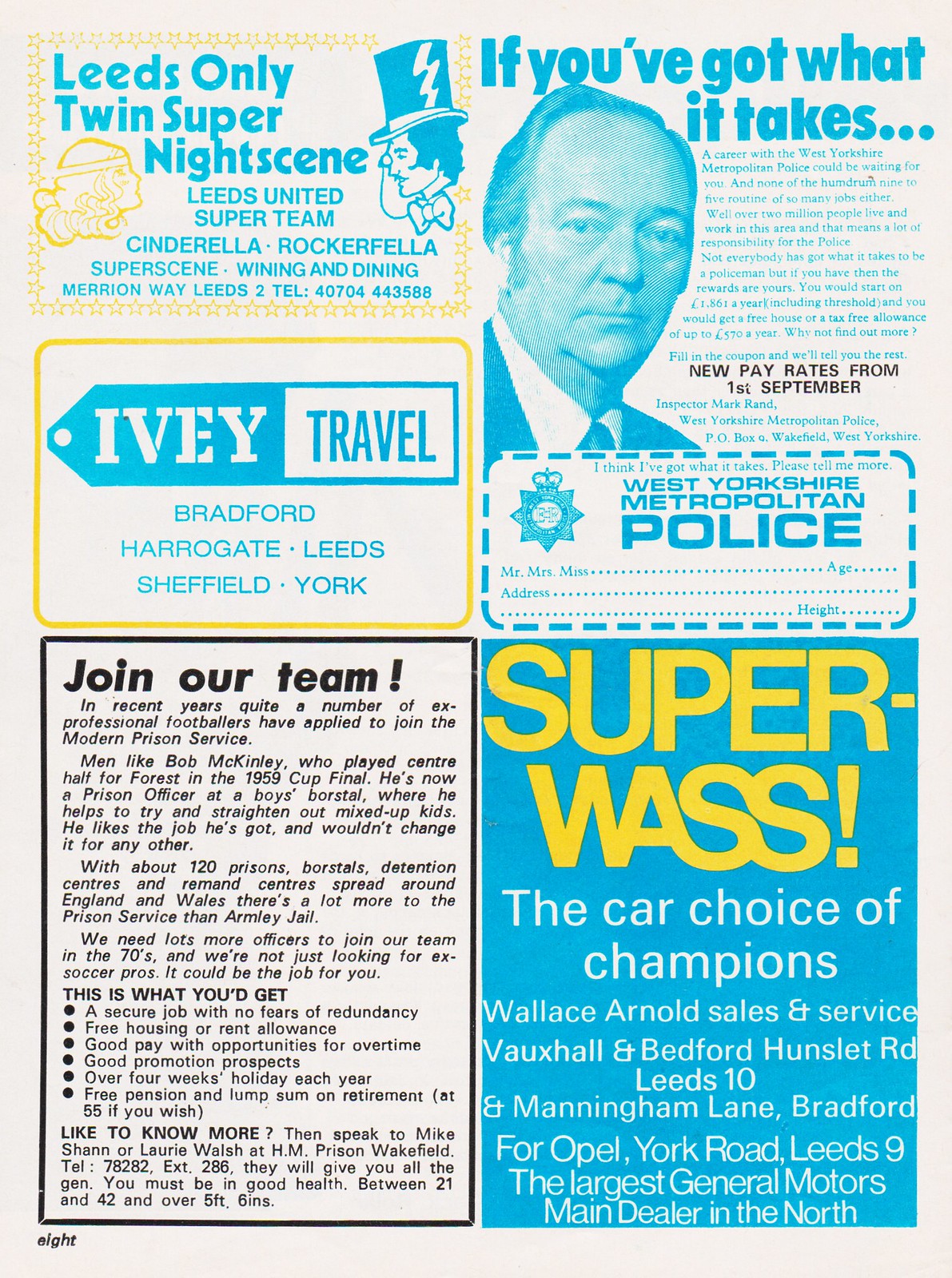The image is a scan of a magazine page divided into four main sections filled with a mixture of advertisements and recruitment notices. The top-left section prominently features an ad with the phrases "Leeds Only, Twin Super, Night Scene," and includes references such as "Leeds United Super Team" and "Cinderella vs. Rockefeller Super Scene." This section also contains contact numbers and a picture of a man wearing a top hat. Below this, there's another ad in a business card format for "Ivy Travel," listing locations including Bradford, Sheffield, York, and New York.

On the upper right section, there is a recruitment ad by the West Yorkshire Metropolitan Police with the bold blue phrase, "If you've got what it takes," accompanied by an image of a serious-looking man in a suit. Below this, in another business card format, is content in bold black font saying, "Join Our Team," targeting job seekers.

The bottom left section continues with recruitment messaging, specifically for HM Prison Wakefield, also reinforcing the "Join our team" recruitment drive. 

Finally, on the bottom right side, in large bold yellow font, there is an advertisement stating, "Super Bus, the car choice of champions," which appears to promote Wallace Arnold sales and Vauxhall servicing. The page is an intricate tapestry of various ads and notices, primarily utilizing blue and yellow hues for their texts and borders.